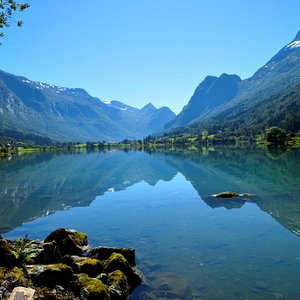This image captures a breathtaking landscape featuring a serene, crystal-clear lake nestled in a picturesque mountainous valley. The lake's pristine blue waters reflect the azure sky and towering mountains that surround it, creating a mirror-like effect. The skies are completely clear, with no clouds in sight, enhancing the tranquil nature of the scene. 

Lush greenery, possibly including dense patches of trees, borders the lake. These verdant areas extend up to the rugged mountains, which rise majestically in the background. The peaks of these mountains are capped with glistening snow, adding a touch of contrast to the vibrant greens below. 

On the right side, a dense forest climbs the mountain slopes, creating a scenic blend of natural elements. In the foreground, the lake's crystal clarity reveals several gray rocks covered in soft, green moss in the bottom left corner, lending a touch of texture to the landscape. Nearby, an object with a greenish hue juts out from the water on the right side, its form indistinct but possibly also adorned with moss.

The lake's surface mirrors the stunning surroundings, reflecting the snow-capped peaks and verdant mountainsides, contributing to the overall sense of harmony and beauty. From the top left, a few green leaves are visible, suggesting that the photo might be taken from a vantage point near a tree. Overall, the scene exudes a sense of peacefulness and natural splendor on a perfect, clear day.